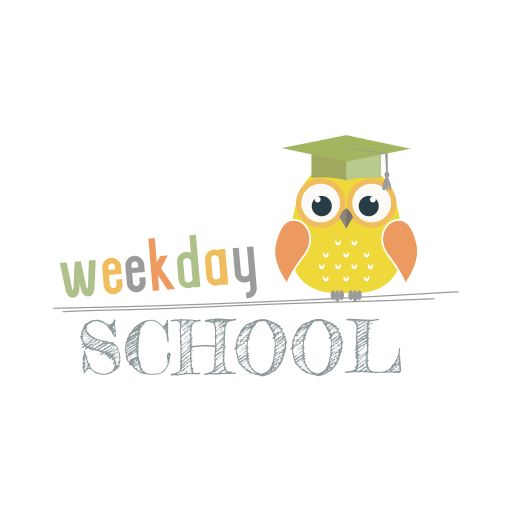The image is a digital graphic set against a solid white background. At the center, the word "weekday" is displayed in colorful, lowercase letters. The W is green, the first E is yellow, the second E is blue, the K is red, the D is green, the A is yellow, and the Y is blue. To the right of "weekday," there is a brightly colored owl, which is looking directly forward and is adorned with a green graduation cap that has a gray tassel. The owl features orange circles around its eyes, orange wings, a yellow body, white specks on its belly, and gray talons. Below "weekday" and the owl, a line is drawn, and underneath this line in large, gray, capital letters is the word "SCHOOL." The composition appears to resemble a logo or icon likely intended for an educational website, with the text and owl centrally positioned with some emphasis on visual balance and color coordination.